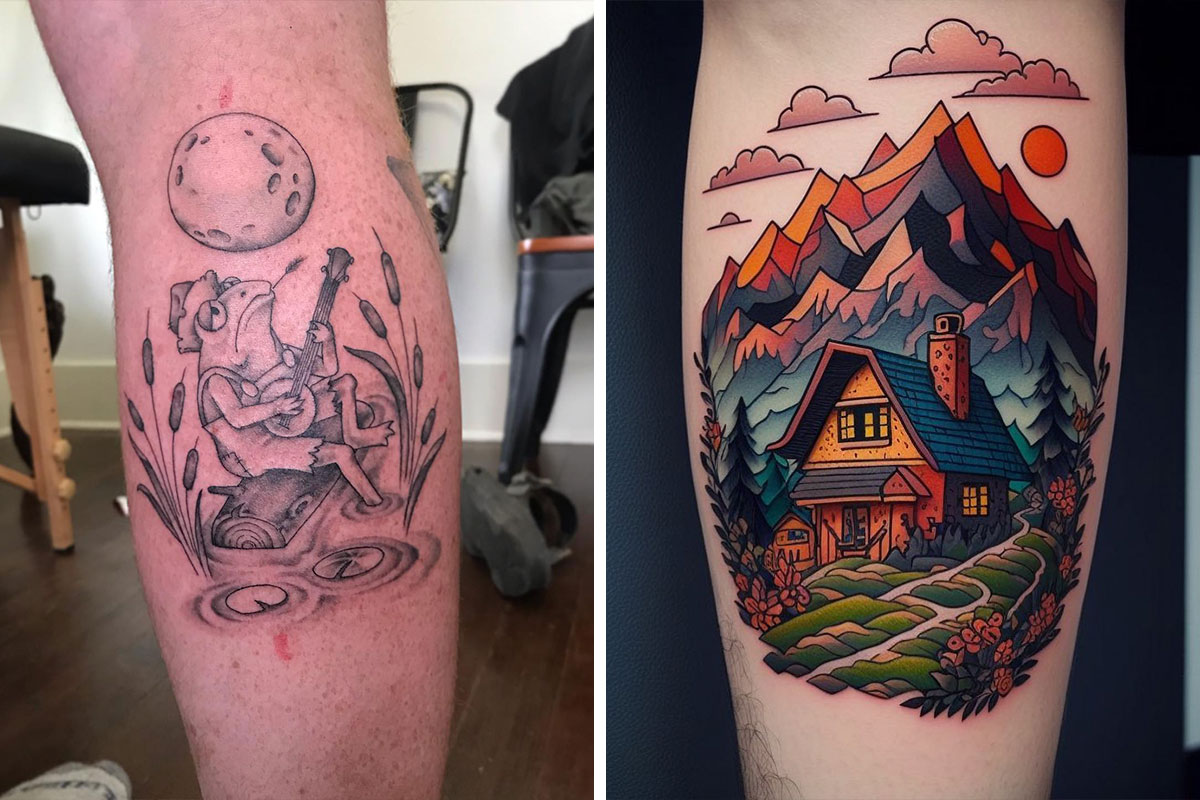This image showcases two photographs side-by-side, each depicting elaborate tattoos on a person’s body, likely on their calves. The tattoo on the left features a highly detailed black ink illustration of a sad frog seated human-like on a log in a pond, with its right leg dipped in water amongst lily pads and pond fronds. The frog, wearing glasses, a hat, and tattered clothing, plays a banjo while chewing on a piece of wheat grass and gazing up at the moon. The background of the scene includes white walls, a black chair on the right, and a wooden floor. The tattoo on the right displays vibrant, colorful artwork of a quaint two-story house with blue roofs and a chimney, nestled in a hilly environment with trees, green grass, and a garden. The setting includes mountains of blue, red, and black hues, with a yellow sun and clouds adorning the sky. The background behind the right tattoo appears dark, contrasting starkly with the lively scene on the skin.